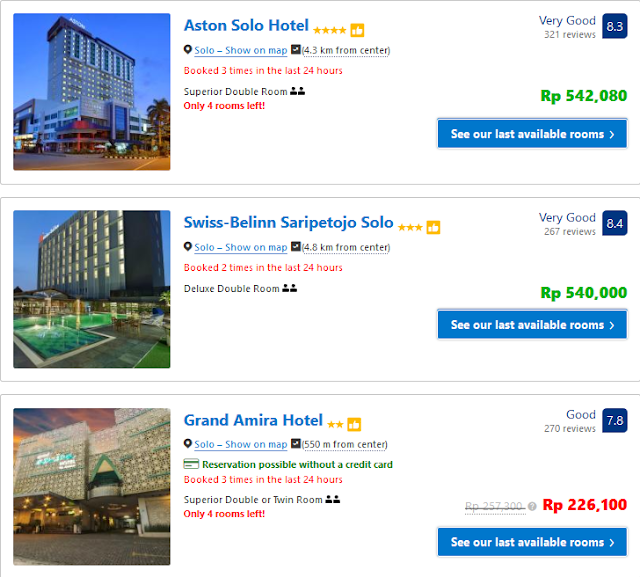Here's a cleaned-up and detailed caption for the described image:

---

Screenshot from a travel booking page displaying three hotels in a vertical list. Each hotel is presented in its own rectangular section. On the left side of each rectangle, there is a thumbnail image of the hotel's exterior or interior. 

In the middle section, the details for each hotel are listed clearly:
1. **Hotel Name** - The first hotel is "Ashton Solo Hotel," which is rated "Very Good" with a score of 8.3. Only four rooms are left.
2. **Swiss Belen Geppetto Solo** - This hotel also has a "Very Good" rating.
3. **Grand Amira Hotel** - This is rated "Good."

Included are:
- Hotel ratings indicated by scores and descriptors like "Very Good" or "Good".
- A clickable "Show on map" option.
- Information on the number of recent bookings within the last 24 hours.
- Room type details such as "Superior Double Room" and "Deluxe Double Room".
- A note on the number of rooms available.

On the right side, the price information is displayed along with review highlights that state "Very Good" or "Good" along with the number of reviews. The designation "RP" is noted with associated numbers, some marked in red and others in green, possibly indicating price changes or special offers. The phrase "See our last available rooms" is also mentioned, emphasizing limited availability.